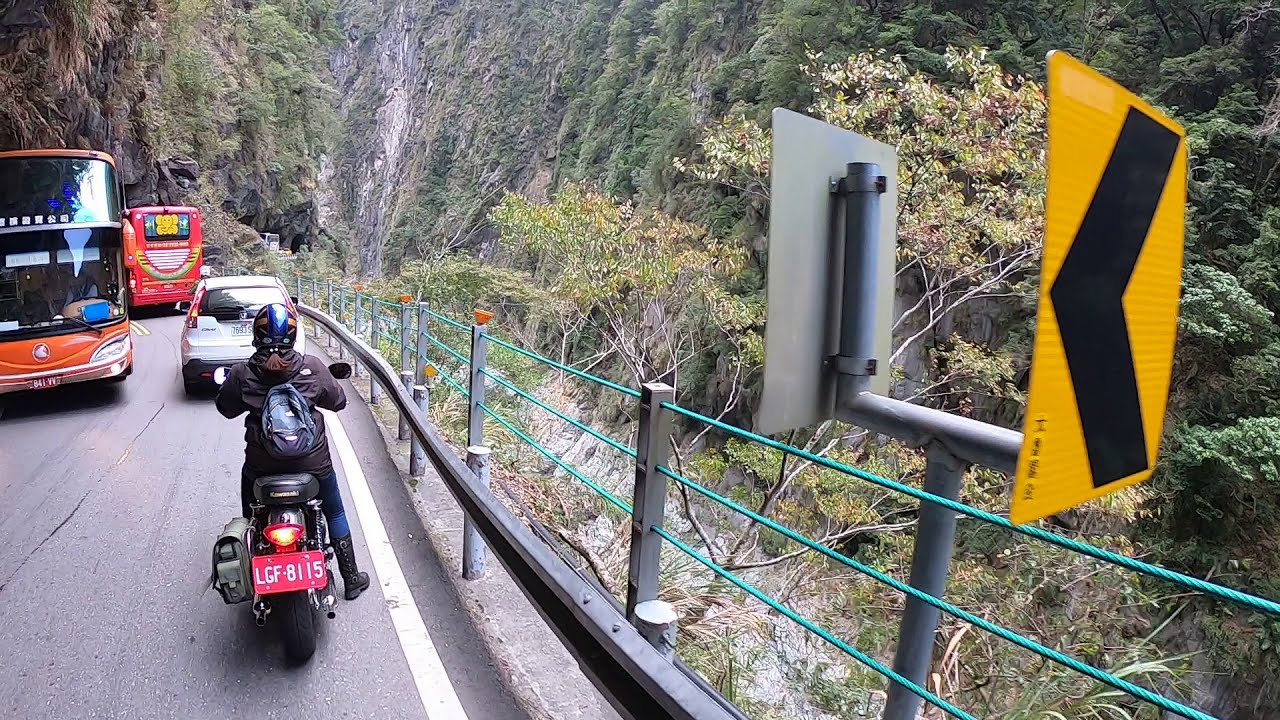In this color photograph, we see an outdoor scene featuring a vibrant highway cutting through a rugged, scenic landscape. The image captures multiple vehicles traveling on a two-lane road flanked by sheer, stony cliffs on both sides. In the right lane, closest to the viewer, is a motorcycle ridden by a woman wearing a helmet and a backpack, with a red license plate reading LGF-8115. Ahead of her is a white Honda sedan, which is closely followed by a red bus navigating a curve. To the left, an oncoming orange double-decker bus, possibly with two children on board, approaches. The highway is bordered on the right by a guardrail supported by green horizontal wires and wood posts, beyond which the terrain sharply descends into a valley. A yellow traffic sign with a black arrow indicates a curve ahead, contributing to the scene's navigational context. The landscape is enriched by scruffy trees and natural rocky formations, creating a picturesque yet dramatic route that is both visually striking and immersive.